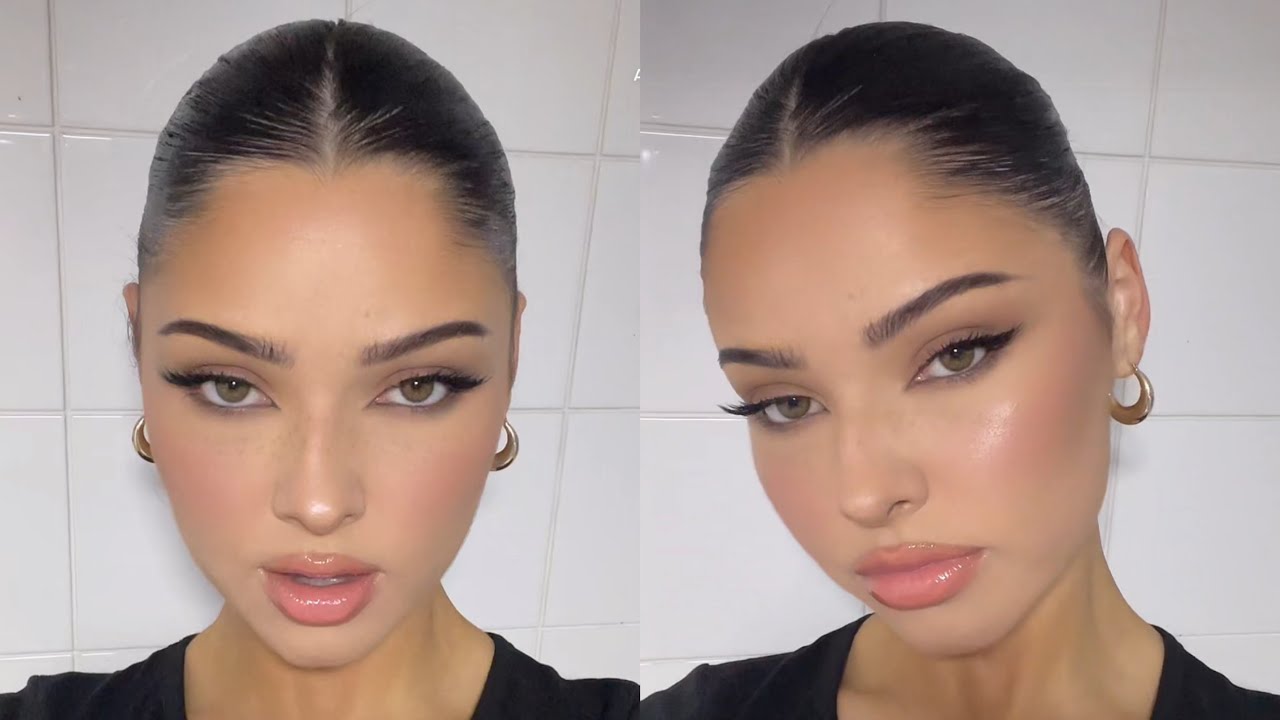Captured in this image is a beautiful young girl against a backdrop of a white towel. In the first picture, her hair is parted down the middle and pulled back, highlighting her stunning brown eyes, which are accentuated with well-applied makeup, making her lashes appear pointed and elegant. Her features include a refined nose and full, nicely shaped lips adorned with a light-colored lipstick. She accessorizes with small gold hoop earrings and wears a stylish black top. In the second picture, she is gazing sideways, showcasing her high cheekbones and overall graceful appearance.